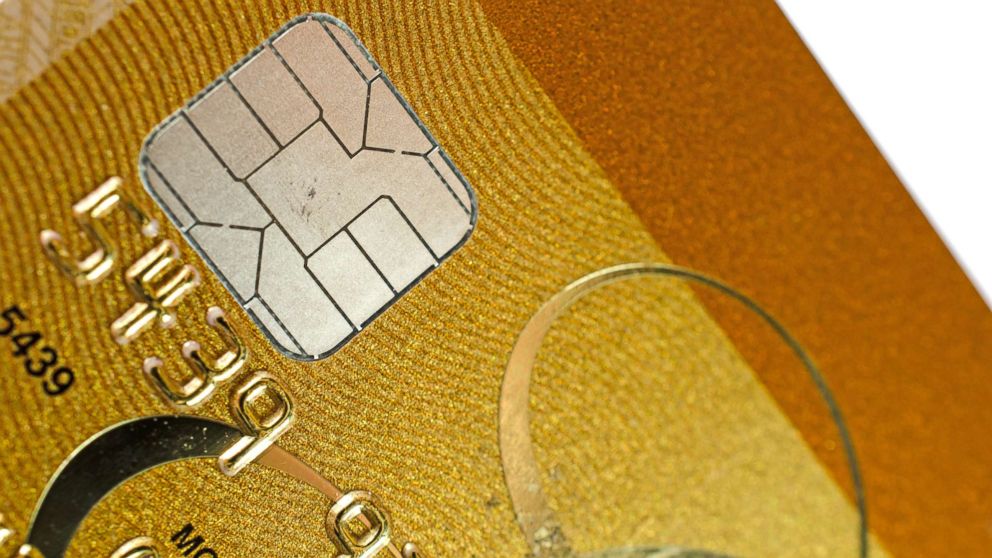This image is an extreme close-up of the left side of a credit or debit card, canted at a 45-degree angle. Dominating the upper left quadrant is a silver microchip with intricate black lines that immediately draw the eye. The card features a mustardy-gold metallic strip along the upper edge, which is glittery and reflective, speckled with fine flecks. Below this strip, the card transitions into a gold background with a fingerprint-like texture formed by thin, wavy, brown stripes. Visible numbers on the card start with "5439," and on the bottom left quadrant, there's a distinctive silver swoop. In the bottom right quadrant, there is a small hoop-like shape that could be part of the card design or something external. The overall texture and shimmer of the card give it a sophisticated, reflective feel.